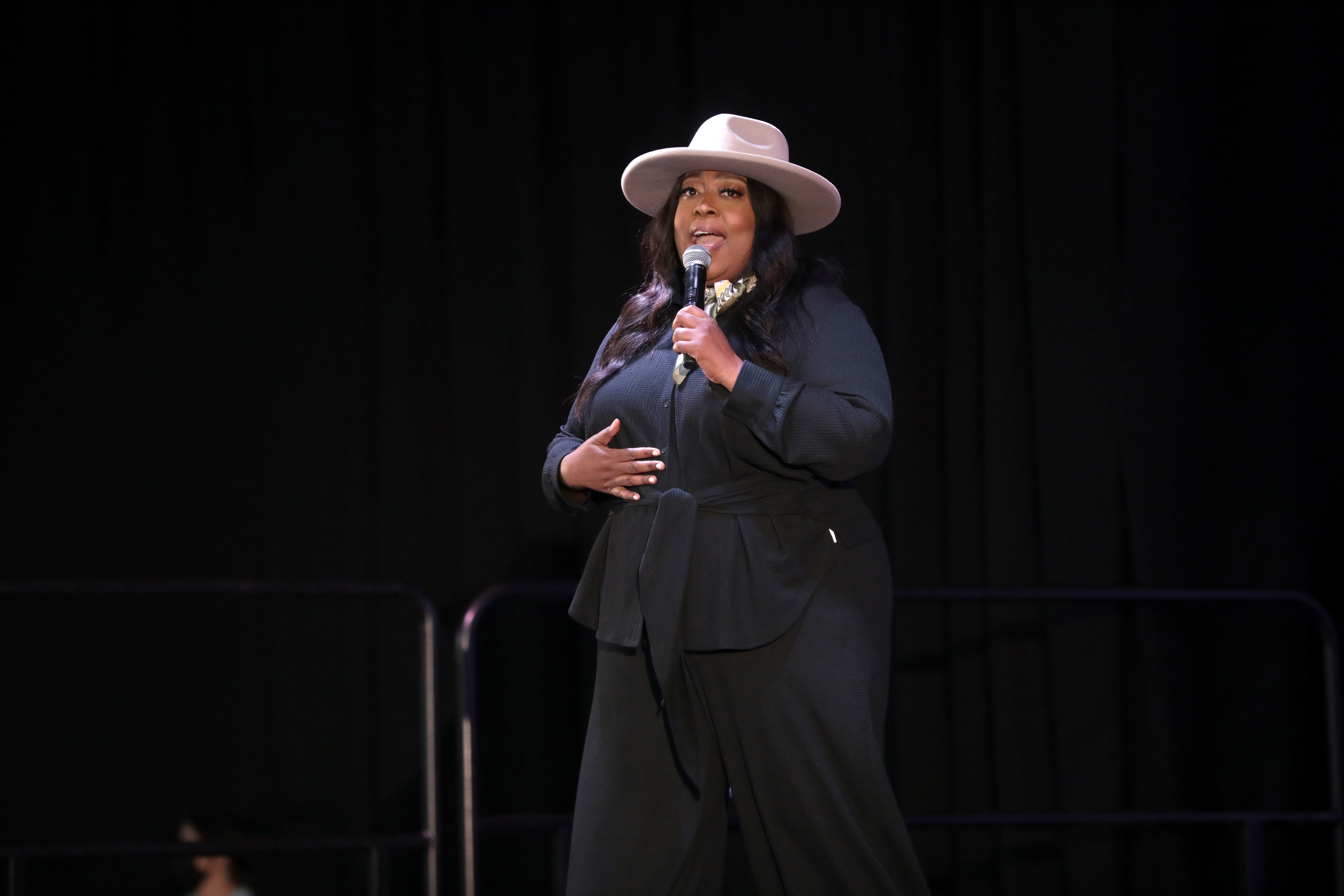The image depicts an African-American woman, slightly on the heavier side, performing on stage. She is dressed in a black ensemble consisting of a long-sleeve buttoned top, which is tied off at the chest, and loose-fitting black pants. She accessorizes her outfit with a white cowboy hat that has a thick, smooth brim, covering her forehead and stopping just above her thin, horizontal black eyebrows. Adorning her neck is a scarf with a white and black color pattern. Her long, wavy black hair flows out from under her hat. In the image, she is holding a microphone with her left hand up to her open mouth, revealing the bottom part of her top teeth and a light pink tongue, suggesting she is in the midst of speaking. Her right hand rests over her stomach. The background features a black curtain and a silver microphone stand is visible to the bottom left of her, placing her in a performance setting, possibly in front of an audience.